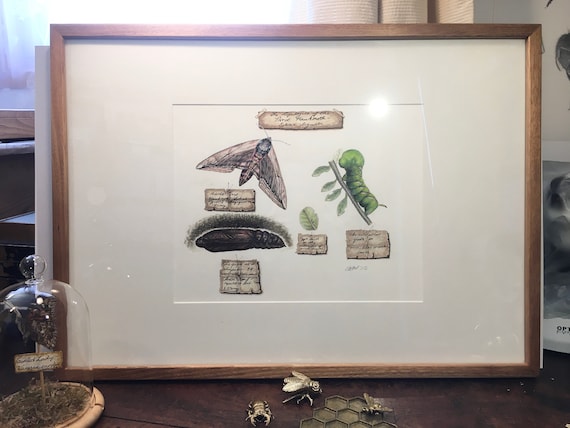The photograph captures a dark wooden desk with various intriguing objects arranged on its surface. Dominating the scene is a framed picture adorned with light honey-colored wood, leaning against the wall. This picture showcases detailed paintings of caterpillars, moths, larvae, and leaves. Below this picture, arranged meticulously on the desktop, are small sculptures of bees crafted from silver, along with a small honeycomb sculpture adding to the theme.

To the left side of the desk, there's an elegant glass dome encasing some grass and a petite sign. Just adjacent to this dome, a butterfly is preserved, enhancing the naturalistic display. Behind the entire setup, a brown curtain provides a backdrop, complementing the earthy tones of the frame and desk, thus enriching the overall aesthetic of the composition.